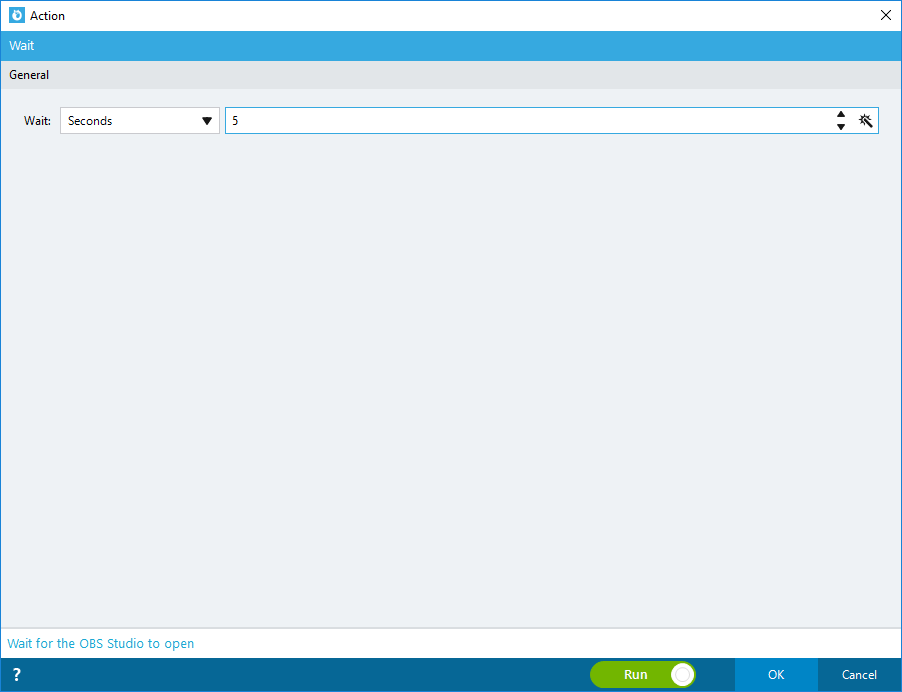The webpage features a light blue background. At the top, there's a white banner with the word "Action" in black text situated in the far left corner accompanied by a blue and white icon. Below this, a medium blue banner showcases the word "Wait" in white letters on the left side. Following that, a gray banner contains the word "General" in black text in the left-hand corner.

The majority of the screen remains light blue and is completely blank. On the primary section of the screen, the top left corner reads "Wait:" in black text, accompanied by a dropdown menu for selecting a time unit beginning with seconds. Adjacent to this is a search bar featuring a numerical dropdown set to the number five.

At the bottom of the screen, a white banner spans across with the phrase "Wait for the OBS Studio to open" written in blue. Directly below, the lowest banner is medium blue. On its left corner, there is a white question mark, and on the right corner, a sequence of elements includes a green on-off switch set to "Run," a green button with the word "Run" in white, followed by a light blue box labeled "OK," and a button labeled "Cancel."